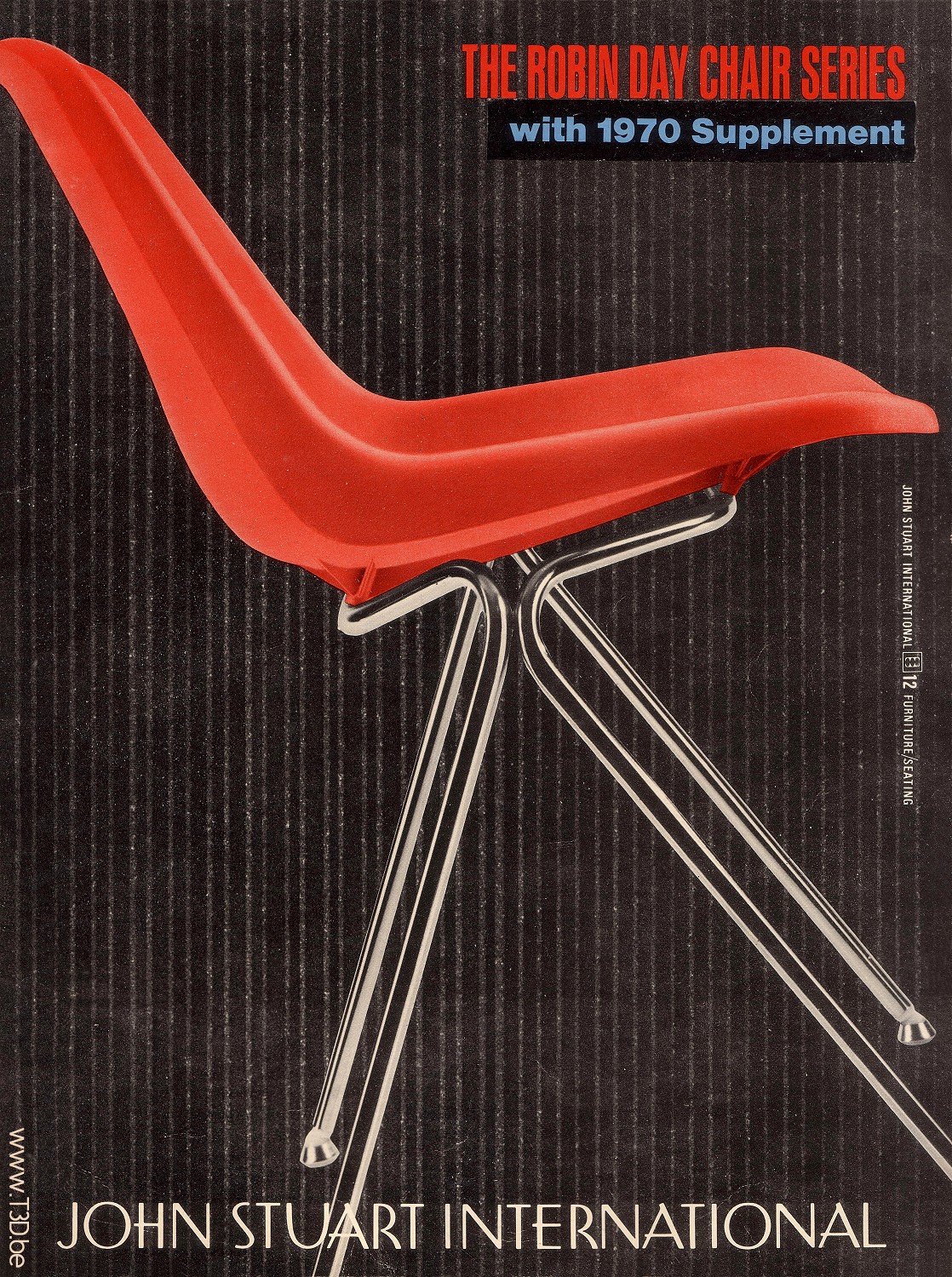The image appears to be an advertisement or catalog cover for a chair series. Dominating the scene is a bold red plastic chair with a sleek, modern design that includes stainless steel legs. The chair spans prominently from the top left to the bottom right, drawing immediate attention with its vibrant color and substantial size. The background features a dark, pinstriped pattern with vertical gray stripes that appear soft and blurry, creating a contrasting backdrop that makes the chair stand out even more.

In the top right corner, red text reads "The Robin Day Chair Series," with a small black bar beneath it containing blue text that says "The 1970 Supplement." The bottom of the image displays the text "John Stewart International" in white. Additionally, small print on the middle right reads "John Stewart International, 12 Furniture / Seating." There is also a vertically positioned URL, "www.t3d.be," located along the bottom left corner. The main colors in the image are red, silver, and shades of gray, with the brownish pinstriped background completing the aesthetic.